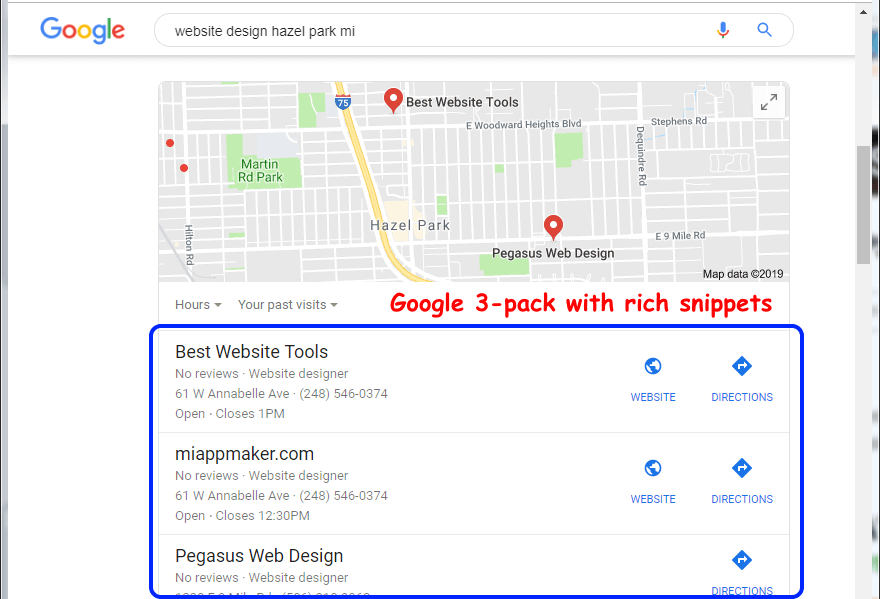The image captures a screenshot of a Google search results page for "Website Design Hazel Park MI." In the upper left-hand corner, the Google logo is prominently displayed. The search bar in the center includes both a microphone icon and a search icon.

The main section of the image showcases a map with a gray background, featuring two location pins labeled "Pegasus Web Design" and "Best Website Tools." Interstate 75 is visible running through the map, along with various white side streets.

Below the map, the text "Google 3-pack with rich snippets" is prominently featured in large red print. Following this, a blue-outlined box contains detailed listings for the two highlighted businesses. 

- "Best Website Tools" includes clickable options for both its website (miappmaker.com) and directions.
- "Pegasus Web Design" offers only a clickable link for directions, with no website available.

Both listings conspicuously lack user reviews, as noted underneath each entry.

The background indicates this Google page is a pop-up, partially overlaying other computer pages, evidenced by partial black-and-white images on both sides.